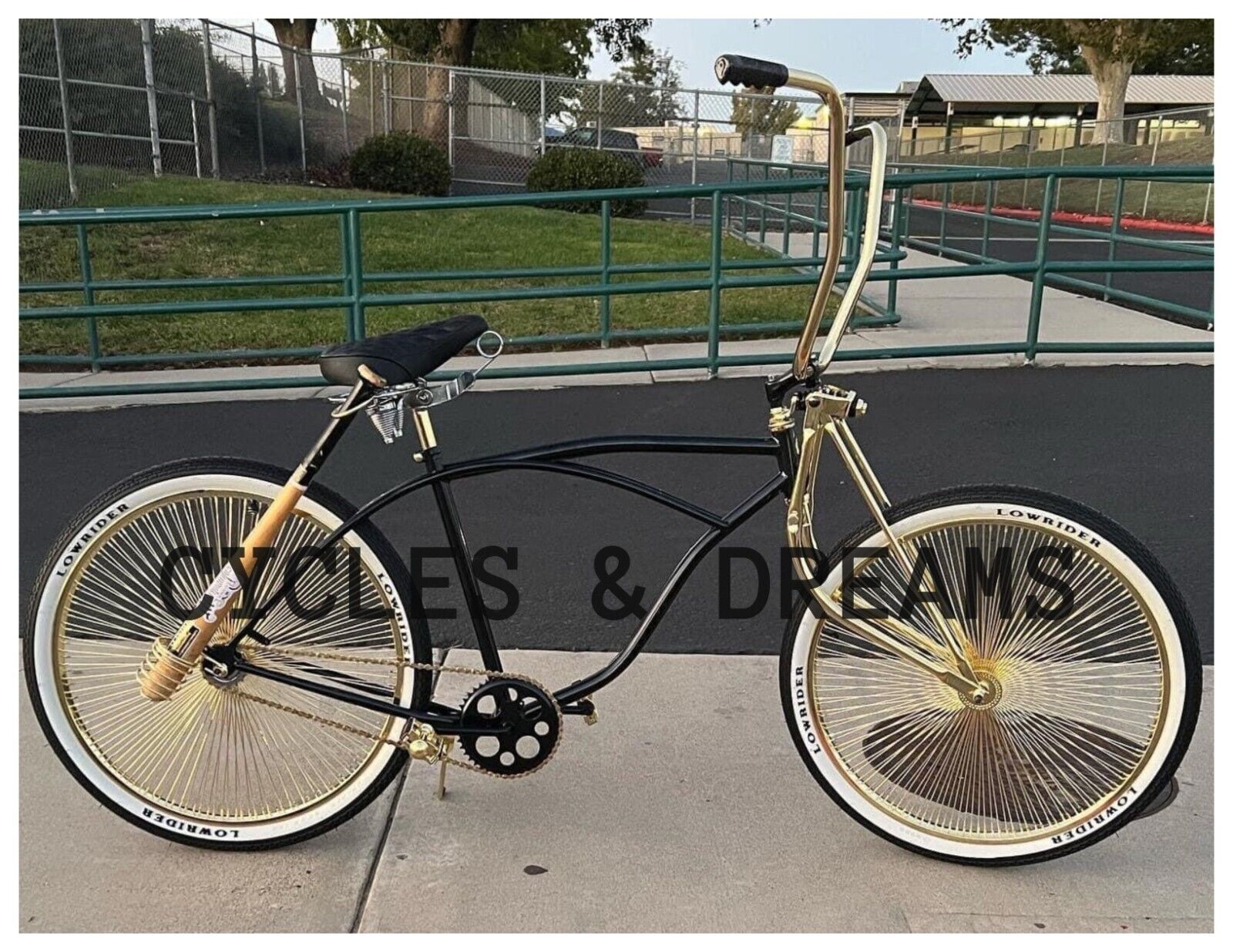This color photograph captures an intricate Lowrider bicycle designed by a Lowrider enthusiast. The bike features a striking combination of black metal and silver chrome for the frame, with numerous gold-colored spokes on the wheels and a gold front fork. The tall handlebars and pedals also display a golden hue, adding to its unique appearance. Adorned with white-wall tires that proudly display the word "Lowrider" in three different spots, the bike exudes a retro charm.

A distinctive feature of this bicycle is the baseball bat mounted from the back wheel to the seat, held in place by a spiral cage-like structure on the side of the wheel. The seat is black, complementing the overall color scheme. Above the bike, the image is overlaid with black text that reads "Cycles and Dreams."

The background reveals an access ramp with green banisters, suggesting the location might be a school or park area. You can see a chain link fence, patches of grass, and buildings in the background, with the sky indicating daytime and the sun low in the sky. This detailed description encapsulates the intricate design and setting of the unique Lowrider bicycle.